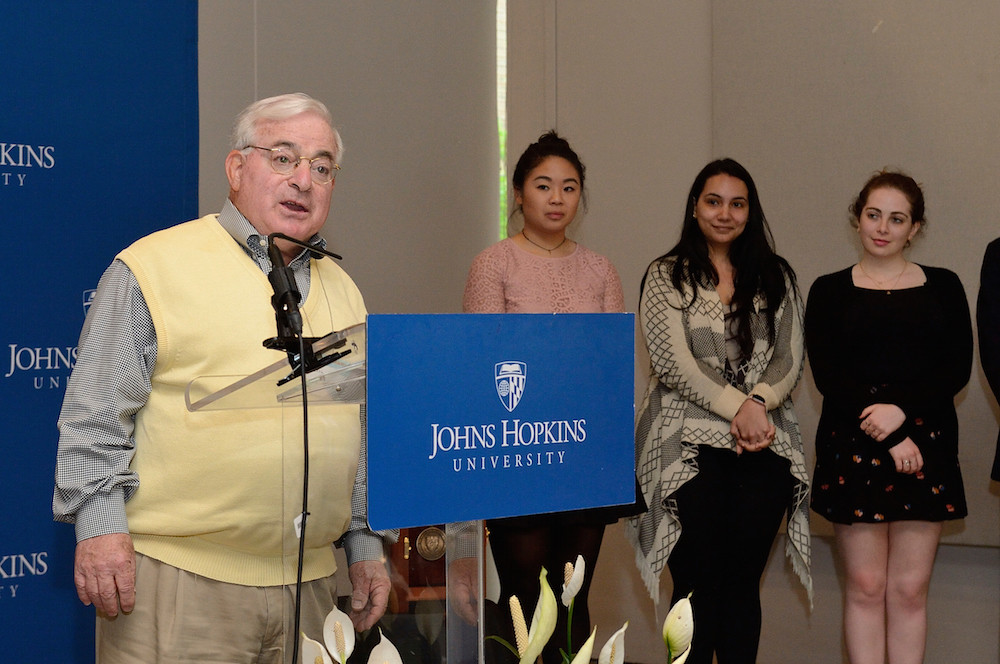In this photograph, an older man with grayish-white hair and glasses is speaking at a clear glass podium adorned with a sign that reads "Johns Hopkins University" in white text on a blue background, partially cut off at the top displaying just "Kins" and "TY." The man, slightly heavy with a round face, is dressed in a yellow vest over a long-sleeved black and white checkered button-down shirt and tan pants. He stands before a microphone as he addresses the audience. The stage is set against a white wall, and there are flowers arranged in front of the podium. Flanking the speaker are three young women, possibly high school or university students, standing in a row. One woman wears a pink shirt, another a long sweater with black pants, and the third a short black skirt. They are all nicely dressed and aligned side by side, with additional text and symbols from the sign obscured by their presence.